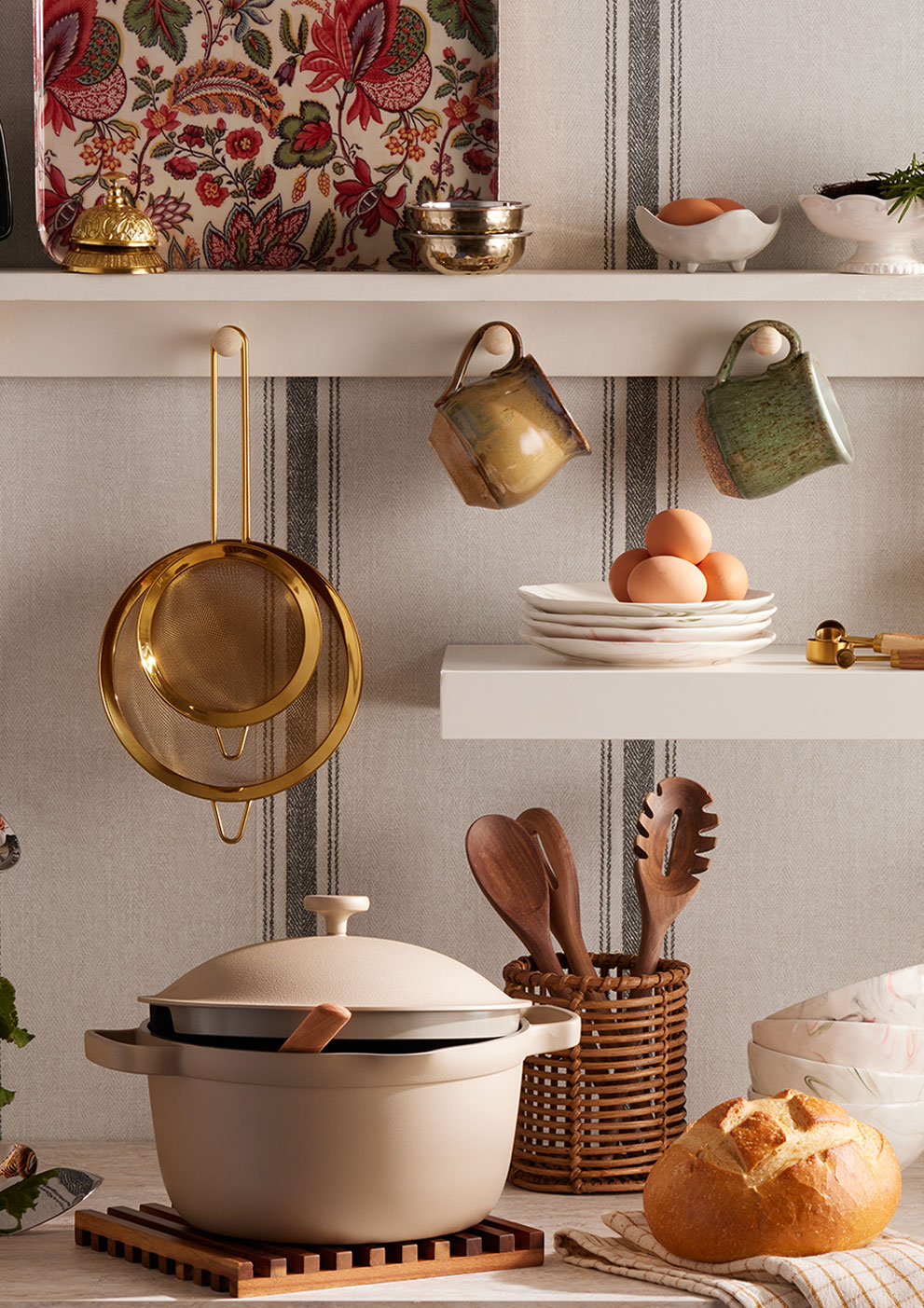This image captures a cozy and detailed kitchen scene, featuring a light wood countertop adorned with various kitchen essentials. A cream-colored pot with a lid rests on a wooden trivet, while a loaf of sourdough bread sits on a beige kitchen towel nearby. A wicker utensil holder contains three wooden spoons, adding to the rustic charm.

Above the countertop are two shelves, set against a wall with white and gray striped wallpaper that mimics a fabric texture. The lower shelf, painted white, holds four white ceramic plates with four eggs, alongside a set of gold measuring spoons. The upper, longer shelf has three knobs hanging beneath it. Two gold strainers dangle from one knob, and a yellow mug and a green mug hang from the other two. This shelf also displays a floral tray with red and green patterns, a gold bell, and two smaller silver bowls stacked together. A white porcelain basket with two orange fruits and a matching pedestal dish with herbs add decorative touches.

Overall, the setting is both functional and aesthetically pleasing, blending utility with charming, country-style decor.